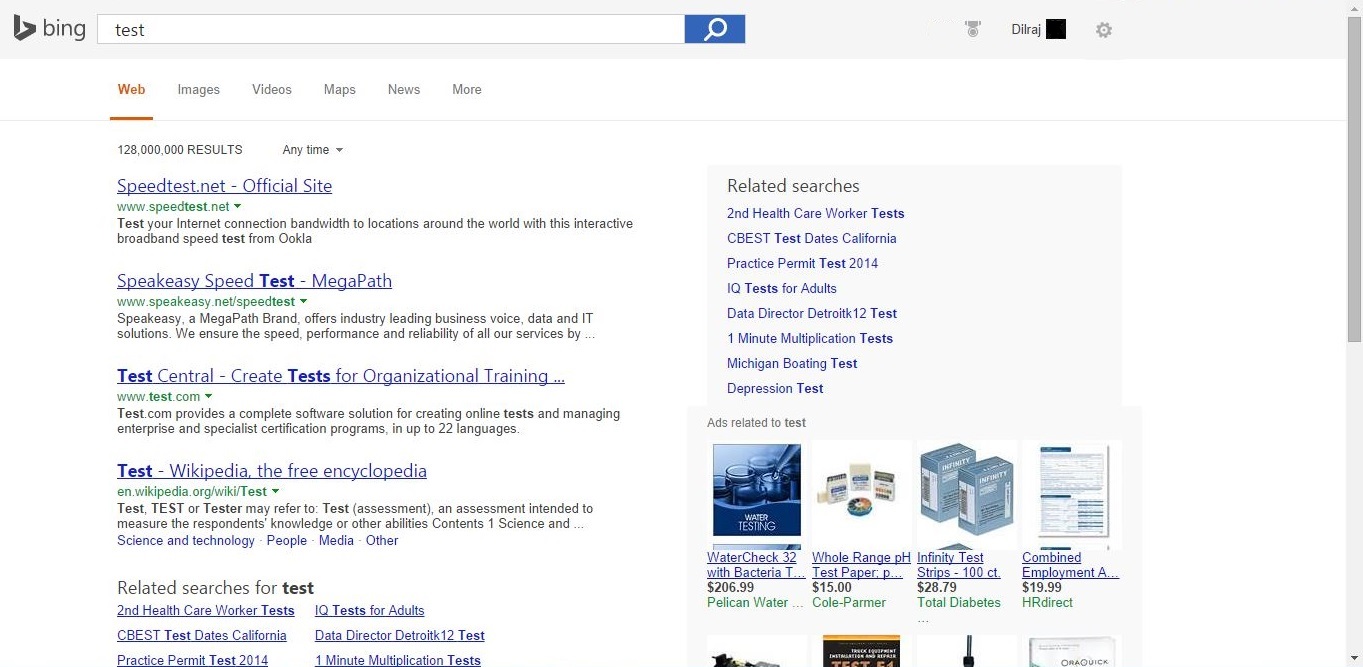This detailed description encapsulates the elements of a Bing search results page for the search term "test."

---

**Image Description: Bing Search Results Page for "test"**

The image features a Bing search engine results page displayed in a landscape rectangular format, approximately twice as wide as it is high. Across the top, there is a light gray header. On the far left of this header, the Bing logo is visible. The logo consists of an angular, lowercase 'b' followed by the word "Bing" in all lowercase letters, both in gray. Centrally located on the header is a long white search box with the gray text "test" prefilled on the left side. Adjacent to the search box, on the right, is a smaller blue rectangle showcasing a white magnifying glass icon representing the search button. Farther right, there is empty gray space followed by three icons; one of them is labeled "DILRAJ" with a black square to its right.

Below the header is the search results section. The top part of this section lists six navigational tabs in light gray: Web, Images, Videos, Maps, News, More. The "Web" tab is highlighted in an orange-red color with a thick underline, indicating the active tab. The search results indicate a total of 128,000,000 results in large, all-caps text.

Detailed below are the first four search results:

1. **Top Result:**
   - **Title:** Speedtest.net - Official Site
   - **URL:** www.speedtest.net (in green) with a downward green arrowhead.
   - **Description:** Test your internet connection bandwidth to locations around the world with this interactive broadband speed test from Ookla.

2. **Second Result:**
   - **Title:** Speak Easy Speed Test - MegaPath (with 'test' in bold)
   - **URL:** www.megapath.com (in green)
   - **Description:** Two additional descriptive lines.

3. **Third Result:**
   - **Title:** Testcentral - Create Tests for Organizational Training (with 'test' and 'tests' in bold)
   - **URL:** www.test.com (in green)
   - **Description:** Two summary lines followed by an ellipsis indicating more content.

4. **Fourth Result:**
   - **Title:** Test - Wikipedia, the free encyclopedia
   - **URL:** www.wikipedia.org (in green)
   - **Description:** Three descriptive lines of text.

Following the main search results, a section titled "Related Searches for test" is divided into two columns of three blue underlined links each. Examples include "IQ tests for adults" in the top right. To the right of this main content, there is a grayish rectangle labeled "Related Searches" at the top, listing eight additional related search terms in blue font, the last being "depression test."

Further down the page under the "related searches" box, products related to the word "test" are displayed. These appear in a row of four images with another partial row. For instance, the top-left product features a rectangular portrait image with blue shading and is labeled "Water Check 32 with Bacteria T" priced at $206.99, with additional product details in green text.

The right portion of the page returns to a more extensive white background, maintaining the structured yet detailed layout typical of a Bing search results page.